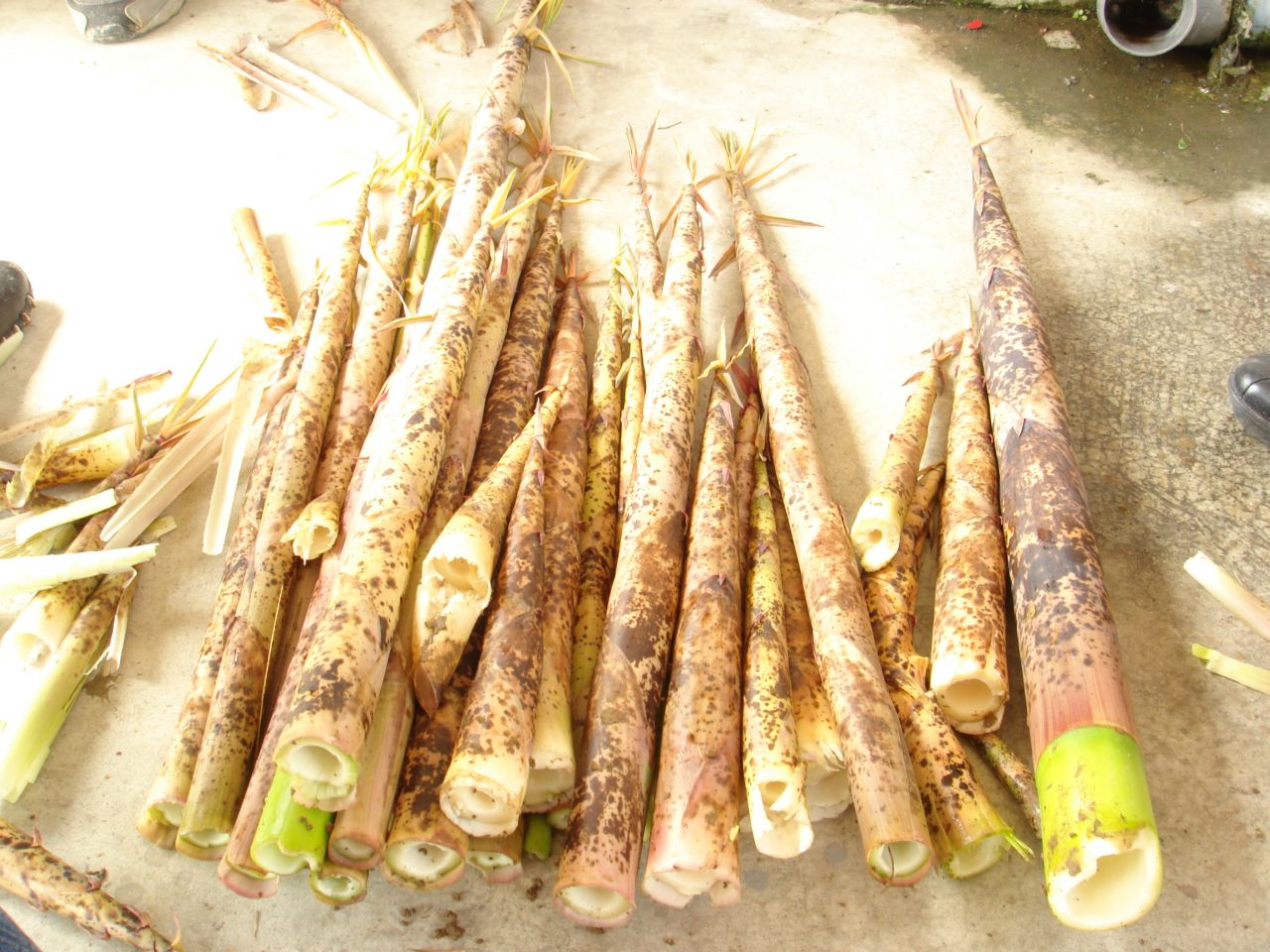This is a colour photograph taken outside, showing several long, tubular vegetable stalks arranged on a dirt or mottled grey surface. The focal point is a pile of these stalks positioned vertically, with their hollow, white interiors and brown, slightly speckled exteriors visible. Some parts of the stalks exhibit a bright green hue beneath the brown skin, particularly near the tapered, cone-like tops where yellowish-green leaves or roots emerge. The scene also features smaller piles of shavings and additional stalks off to the left. In the upper right corner, partially in view, is a grey pipe, casting a large shadow over the area. A couple of indistinct grey and white objects are noticeable on the left and right edges of the image, adding to the outdoor setting's natural, slightly cluttered appearance.